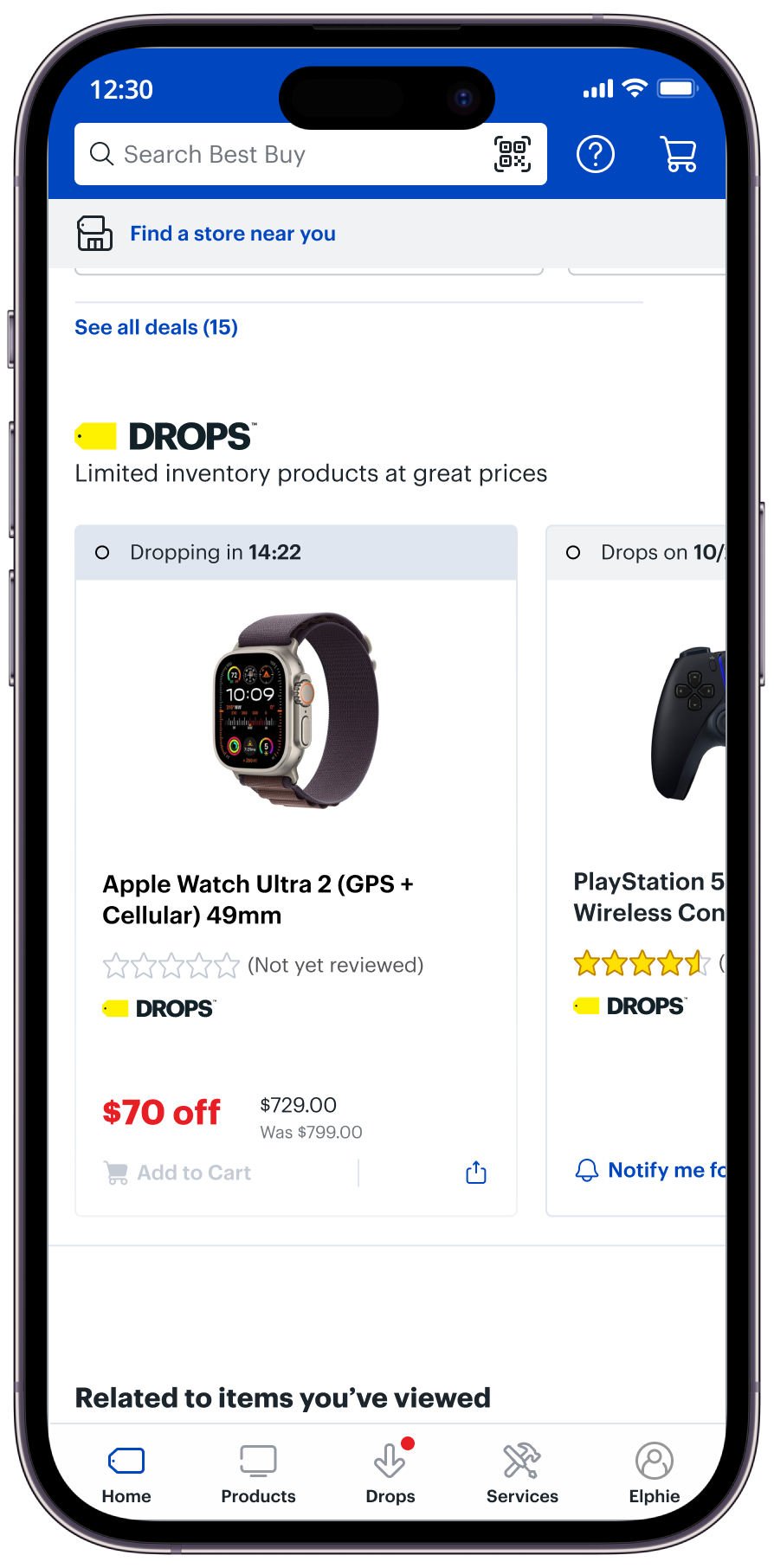This image captures a screenshot of a smartphone displaying the Best Buy website, taken at 12:30 PM. At the top of the screen, there's a white search box displaying the text "Search Best Buy." Below this, a blue hyperlink reads "Find a store near you." 

Dominating the central portion of the webpage is a promotional section featuring a header that reads, "See all deals (15)," followed by the text "Limited inventory products at great prices." Prominently featured in the middle is a product listing for an Apple Watch Ultra 2. This listing includes key details such as "GPS + Cellular" and its size, which is 49mm. Although the listing shows a five-star rating indicator, it notes "Not yet reviewed," signifying no customer reviews have been submitted. 

The price information is displayed clearly: the watch is currently $729, marked in black text, with a red note indicating "$70 off." Directly below, the previous price of $799 is struck through, highlighting the current discount.